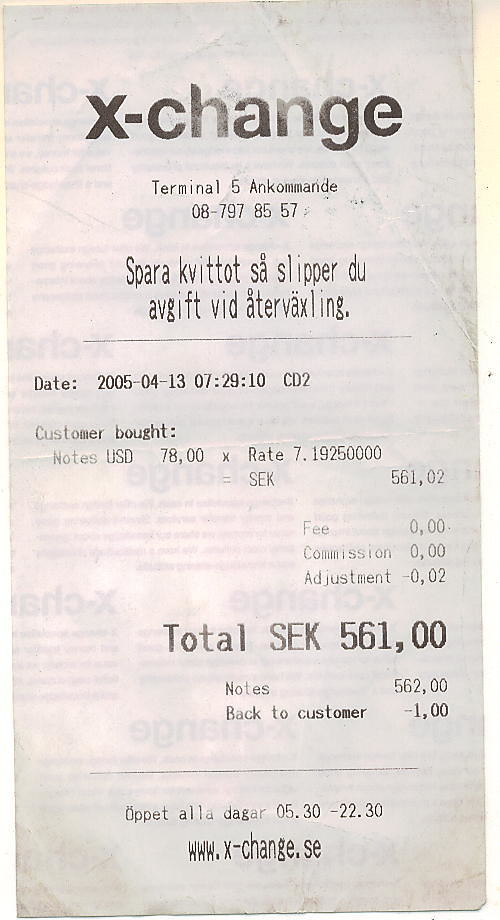This photograph captures a detailed close-up of a receipt set against a slightly overexposed white backdrop, which highlights the paper's texture along with its creases, folds, and scuffs. The top of the receipt prominently features the lowercase word "x-change" in large letters. Directly underneath, in a smaller font, are the details: "Terminal 5, Uncommand 08-797-8557." Further down, the receipt transitions into what seems to be Swedish text. The key information conveyed includes "CustomerBot notes USD 78 times rate 7.1925 equals SEK 56102," indicating a currency exchange transaction where 78 US dollars were converted into Swedish kronor at the specified exchange rate.